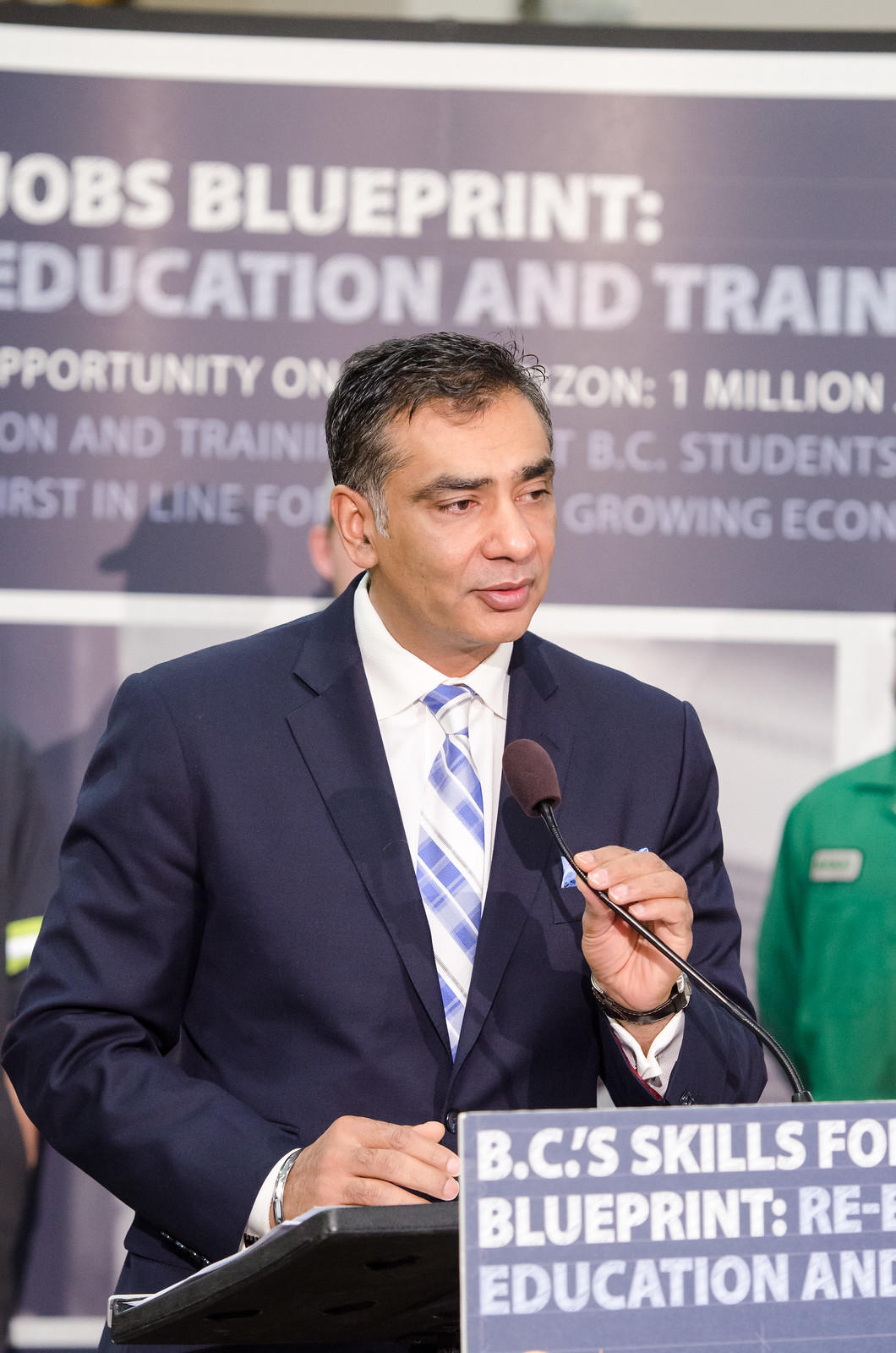The photograph captures a significant moment at what appears to be a political conference or event. The focal point of the image is a well-dressed man of possible Middle Eastern or Indian descent, attired in a dark blue suit accompanied by a white collared shirt and a sophisticated blue and white tie. His appearance is further enhanced with noticeable accessories, including an expensive watch and bracelet. With short, slightly graying black hair, he stands confidently at a podium, holding a microphone between his index finger and thumb, while his other hand rests on the podium. 

He gazes attentively into the audience, ready to address the crowd. Behind him, several observers stand, partially obstructing the background signage which is grey with white fonts. The text on the podium is partially legible, displaying phrases like "BC's Skills," "Blueprint," and "Education." Additional visible words from the backdrop include "jobs," "opportunity," "education and training," "1 million," "BC students," and "growing economy," suggesting the themes of his speech revolve around education and economic growth. The atmosphere of the image points to an official gathering, possibly a rally or a conference aimed at discussing significant societal topics.